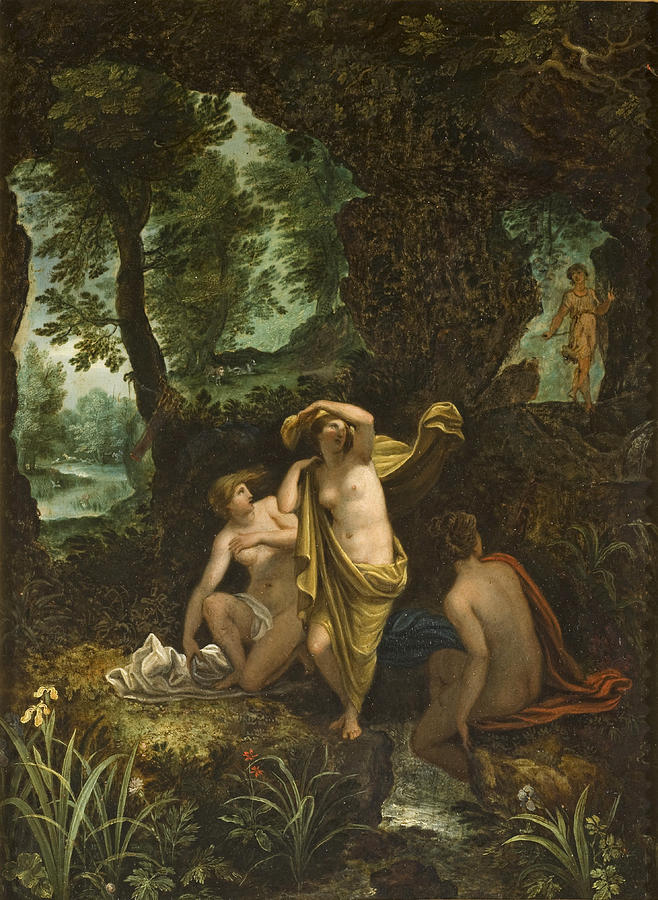This vibrant painting, reminiscent of Roman and Renaissance influences, depicts a lush, green, forested outdoor scene at the edge of a serene, natural wading pool. The classic, realistic style captures three nude women engaging with their surroundings. One woman stands, draping an orange scarf around her shoulder and lower waist, exposing her breasts and stomach. Another woman sits with a yellow-gold wrap barely covering her lower body, while the third, seen from the back, sits with a white sheet loosely over her shoulder. All three women are gazing upwards towards an approaching figure, a clothed woman, walking down a path in the distance. The lush greenery, a river visible far away, and colorful flora, including tiger lilies and yellow lilies, enhance the scene's pastoral beauty, evoking an ambiance of innocent surprise and natural elegance.